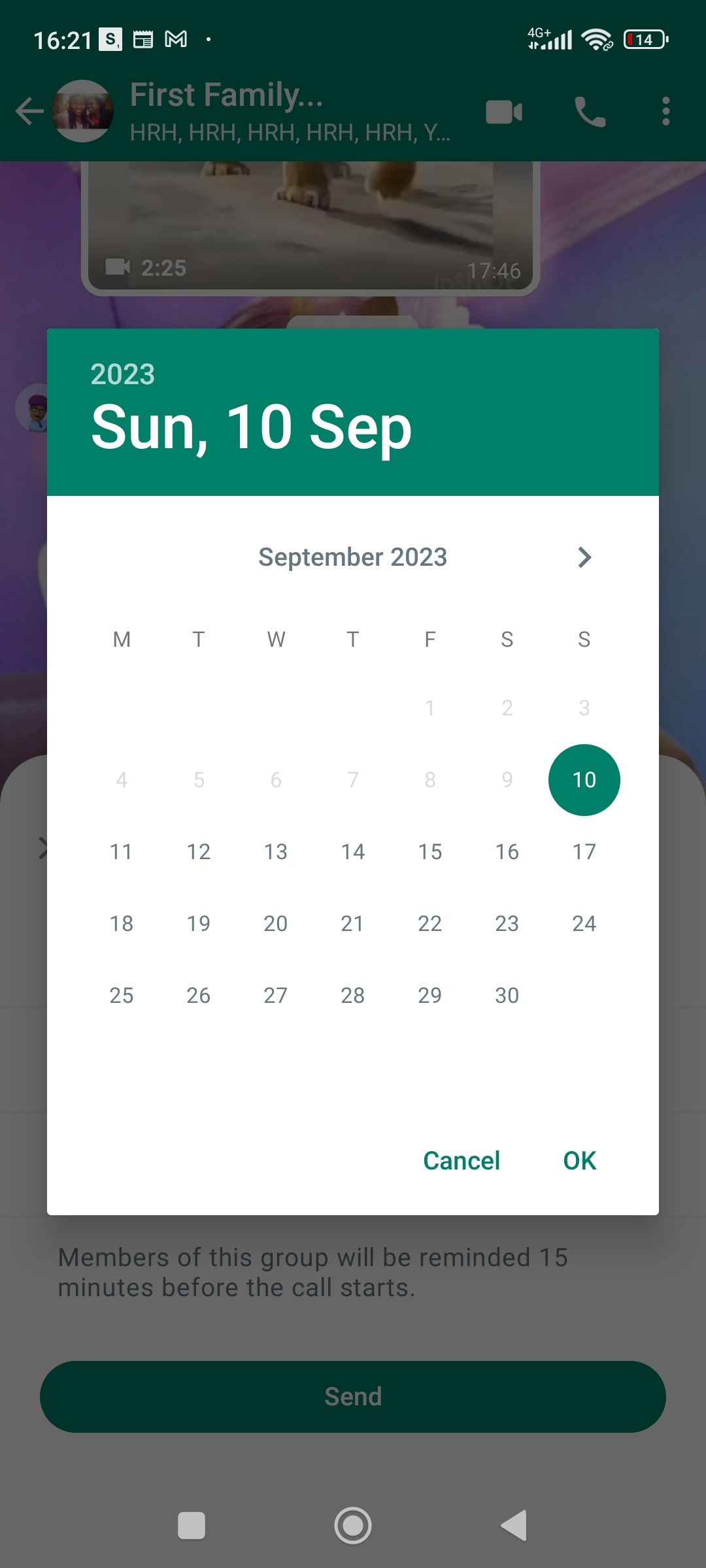This is a detailed caption for an image that is a screenshot in portrait mode. The screenshot features a layered display with a distinct background and an overlaying pop-up chart. 

The primary background shows elements of a smartphone interface. In the upper left corner, the phone's time is displayed as 16:21, while the upper right corner indicates the battery at 14%. Below this, there is a green section that displays an avatar labeled "First Family" with repetitive text "HRH HRH HRH HRH HRH" underneath, the significance of which is unclear.

Overlaying this background is a pop-up chart, specifically a calendar page set against a green background. The top left of the chart displays the year "2023" with the date "Sunday 10 September" directly below. The main body of the calendar, having a white background, shows the month of September 2023 laid out from Monday through Sunday. 

The current date, Sunday, September 10th, is encircled by a green circle, whereas the dates from September 1st to 9th appear grayed out, indicating past days. The upcoming days, from the 11th to the 30th, are displayed in black.

In the bottom right corner of the pop-up calendar are two green buttons labeled "Cancel" and "OK", both designed as clear buttons.

Additionally, the background screenshot shows that the user is interacting with possibly a video or group membership chat, having played 225 minutes out of 1746 minutes in total.